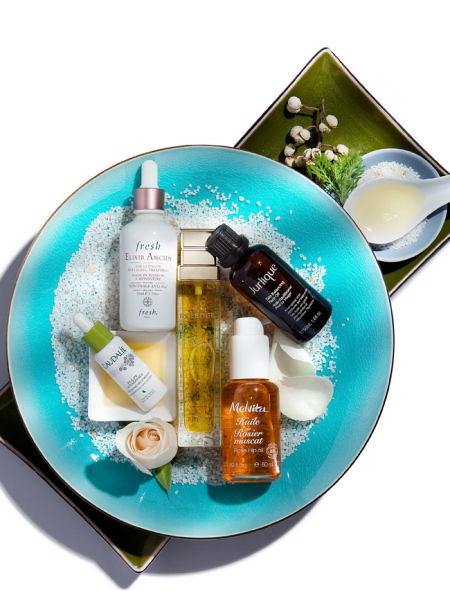The image showcases a meticulously arranged composition on a pristine white background. Central to the arrangement is a green, triangular plate adorned with fresh herbs and delicate white flowers. Adjacent to this plate, a small blue cup filled with powder sits next to a spoon holding a small amount of oil.

Above this setting, a larger blue plate with intricate white and black trim takes center stage. On this plate, a vibrant red rose is prominently displayed alongside a white square bowl containing liquid. Atop the bowl rests a dropper bottle, predominantly white with green accents. Nearby, a petite glass jar with a silver lid, presumably containing a creamy substance, stands next to what looks like a perfume spray and a small white spritz bottle. Additionally, there's an essential oil bottle included in the mix.

Among these items, scattered white rose petals and a mound of finely crushed white substance add to the intricate tableau. Beneath this blue plate ensemble, another green plate with white trim is subtly visible, albeit empty. The arrangement appears to be an assembly of ingredients and tools intended for the creation of a DIY personal care product, possibly for skincare or another personal use.